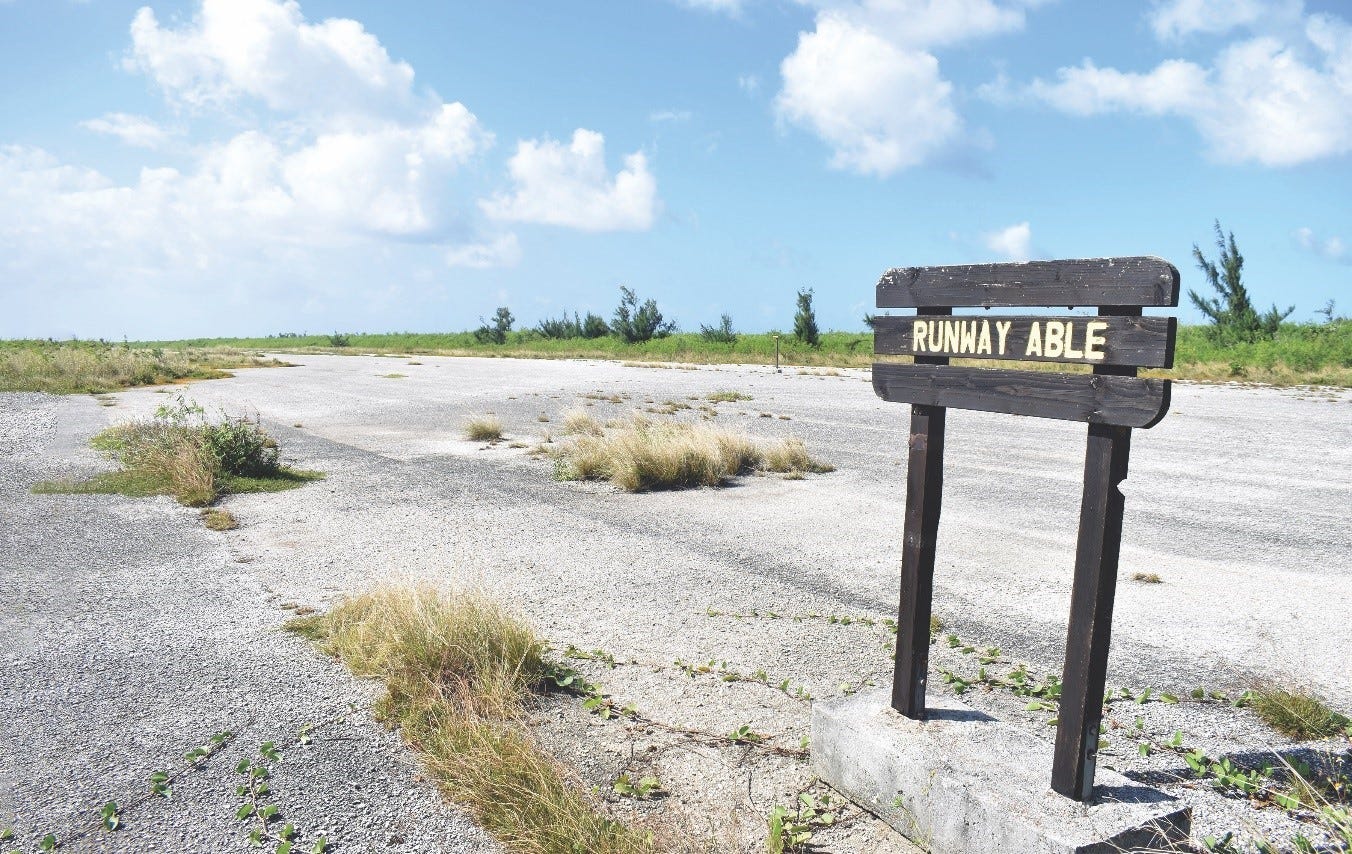The image depicts a desolate, rundown parking lot situated in a remote area, illuminated by the morning sun. The parking lot, which is a faded gray-whitish color likely due to prolonged exposure to sunlight, is marred with numerous cracks from which weeds and grass are prolifically sprouting. Dominating the center of the lot is a substantial patch of weeds, further emphasizing its neglected state. The lot extends towards the left side, where midway up, more grass has emerged. Near the bottom, additional weeds poke through, surrounding a concrete slab to the right. This slab supports a small, weathered wooden sign with three black boards displaying the red lettering "Runway Able." The backdrop features a sprawling field of green grass lining the horizon, dotted with a few sparse trees, all set under a vast blue sky lightly adorned with white clouds, emphasizing the emptiness and forgotten feel of the scene.